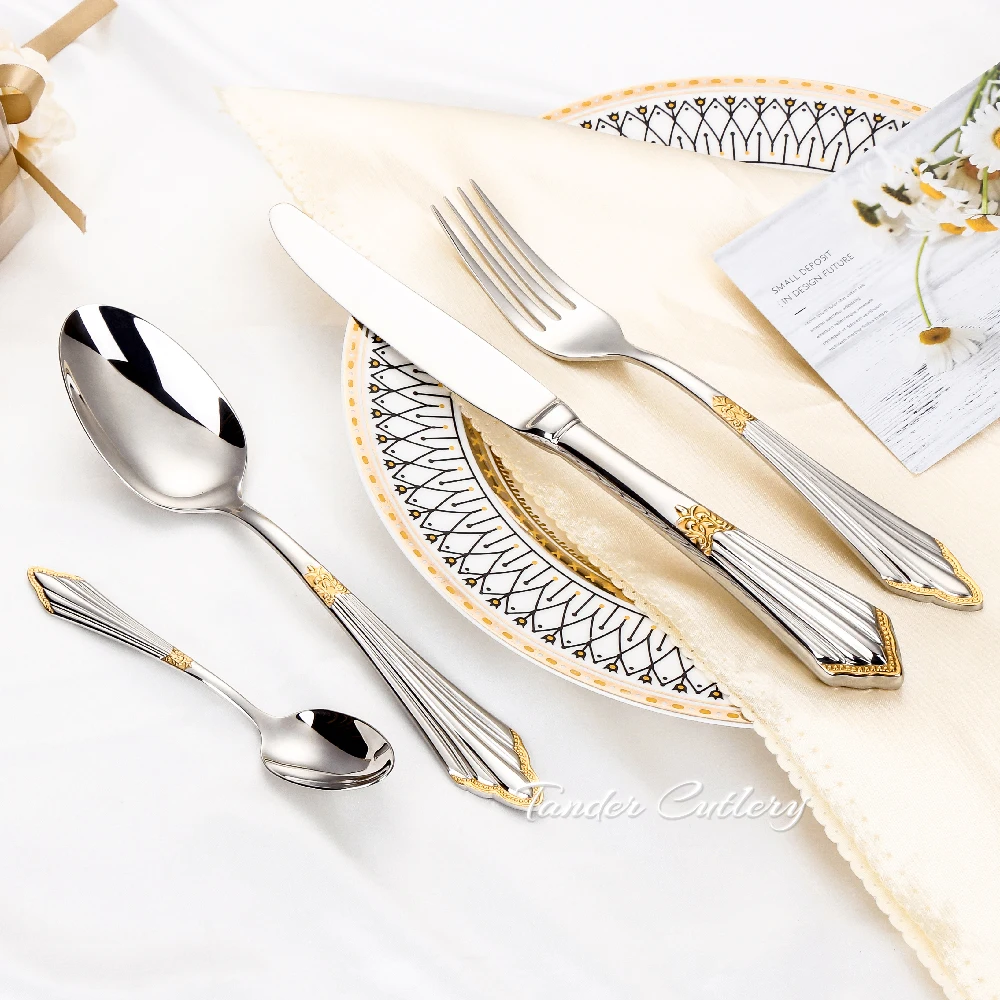The photograph depicts a square-shaped, professionally-taken image of a formal table setting against a bright white, slightly wrinkled tablecloth. At the center of the table setting is an ornate white plate with intricate blue, yellow, and black triangular and arrow patterns along the edge, bordered with gold. Covering the inside of the plate is a light beige linen napkin. Arranged on top of the napkin are a knife and fork to the right, with a large serving spoon and a teaspoon beside the plate. The utensils are made of stainless steel with fluted handles and gold detailing where the handle meets the utensil. Placed at the upper right of the plate is an invitation card featuring a bouquet of daisies and the text "Small Deposit in Design Future." At the bottom right corner of the image, white text reads "Tender Cutlery," suggesting that this photograph might be an advertisement or promotional material for the elegant tableware.